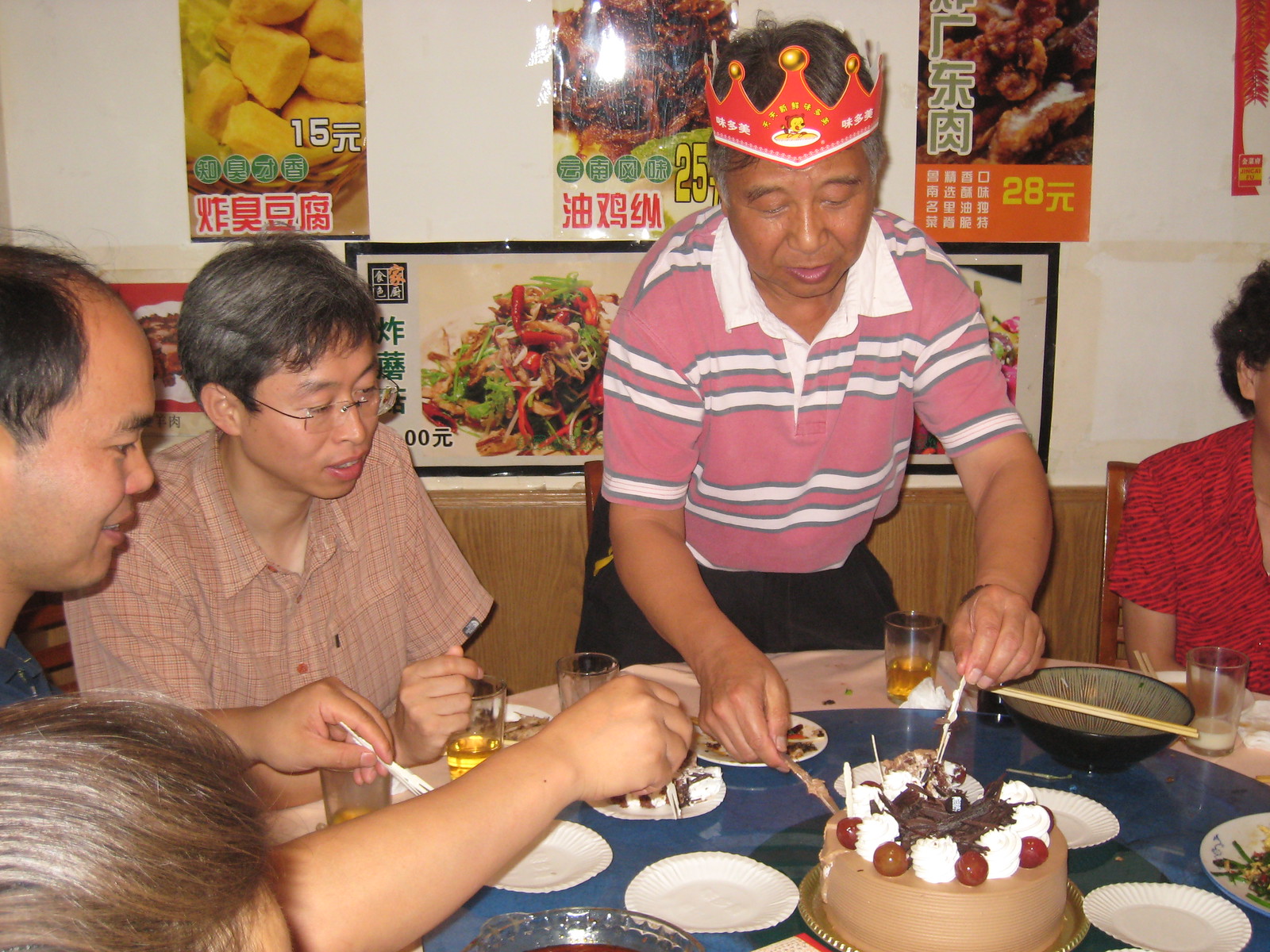In the image, several people are gathered around a circular table in what appears to be a Chinese restaurant, characterized by its white walls adorned with images of various food items and prices, including numbers 15, 18, 25, and 28, along with Chinese characters. The tablecloth is a blue and white pattern, and the table is set with multiple white paper plates, glass glasses, and a bowl with chopsticks. At the center of the table sits a brown cake with red and white circles on top, hinting at a celebration. The individual standing up, a silver-haired older Asian man, possibly in his 50s or 60s, is wearing a red and white striped polo shirt and a red crown. He is in the midst of cutting the cake. The seated individuals around him, also appearing to be older Asians, are dressed in various outfits: one in a red and black ensemble, another in a tan and brown plaid shirt with glasses, and another in a blue shirt. The scene suggests it is someone's birthday celebration, with the man in the red crown likely being the celebrant.